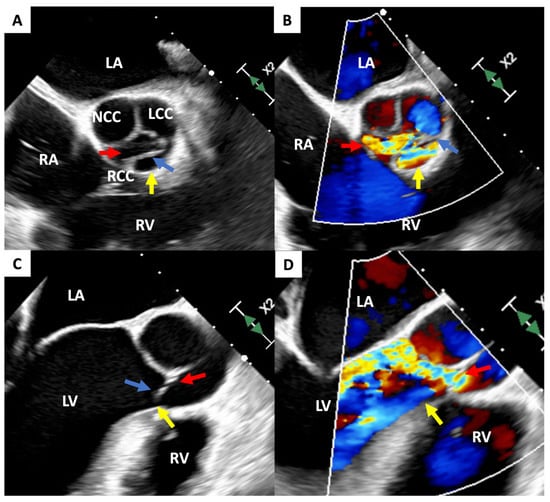The image displays a detailed four-panel digital screenshot of radiology scans, potentially x-ray or ultrasound, labeled A, B, C, and D. The scans feature complex annotations including letters such as A, B, C, D, L, A, N, C, C, L, C, C, R, C, C, R, A, X, 2, R, V, L, V, and various directional arrows in colors red, blue, yellow, and green. Background hues are primarily black and white with overlays of yellow, orange, and more. Each panel highlights specific sections with colored arrows and lines, suggesting focus points, possibly anatomical features or valves. The measurements and indicators, including green arrows marked "X2," add to the detailed analysis provided by the images. The panels show an extreme close-up view of the objects being scanned, though the exact nature of these objects remains unclear.